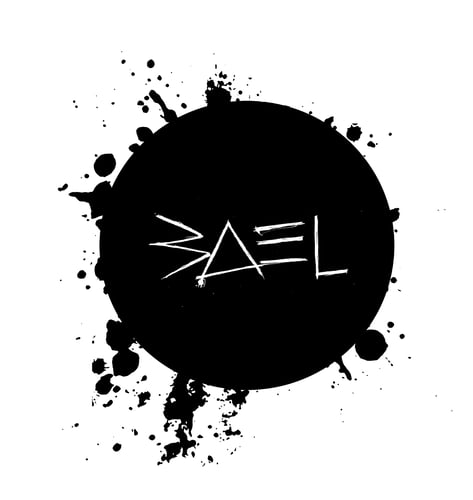The image features a striking black circle at its center, set against a pristine white background. This bold and attention-grabbing circle is surrounded by dynamic ink splatters radiating in all directions, creating a sense of motion and chaos. Within the circle, delicate white text appears almost scratched into the surface, bearing the cryptic characters "B-A-E-L" or "3-A-E-L," alongside other shapes such as a triangle and lines that might suggest additional letters or symbols. The text outside the circle includes a stylized "W" positioned on its side. The entire composition exudes the raw, spontaneous energy of graffiti art, yet it also hints at being a carefully designed logo, possibly intended for a company or brand. The artwork's stark black and white palette further enhances its boldness and simplicity, making it a visually compelling piece.